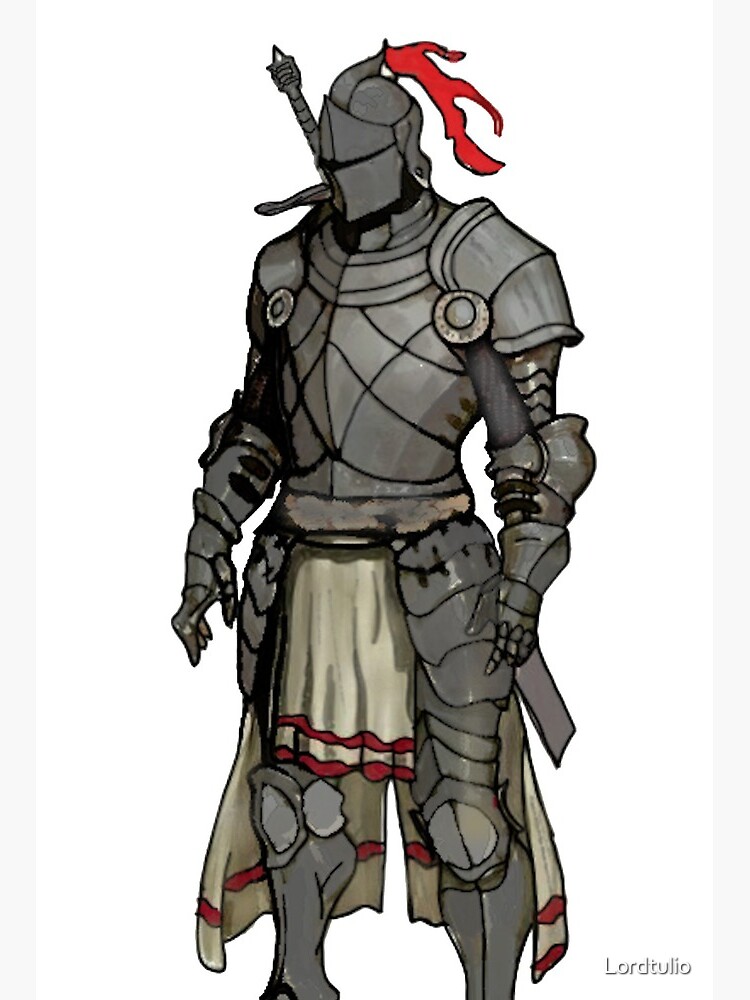This image depicts a digital drawing of a tall medieval knight adorned in full, elaborate armor. Set against a white background, the knight is introduced by the name "Lord Tullio," located at the bottom right of the image. The armor is predominantly metallic gray, encompassing the knight from head to toe, including robust gauntlets and intricate, armadillo-like layering on the legs. Notably, the knight’s helmet, which entirely conceals his face, is topped with a red feather or small flag. The knight also wears a cream-colored cloth piece, akin to a skirt, featuring red trim at the bottom, which is consistent on both the front and back. Adding to the regal appearance is a cape that drapes elegantly from behind. This image captures the strength and nobility typical of iconic medieval knights.